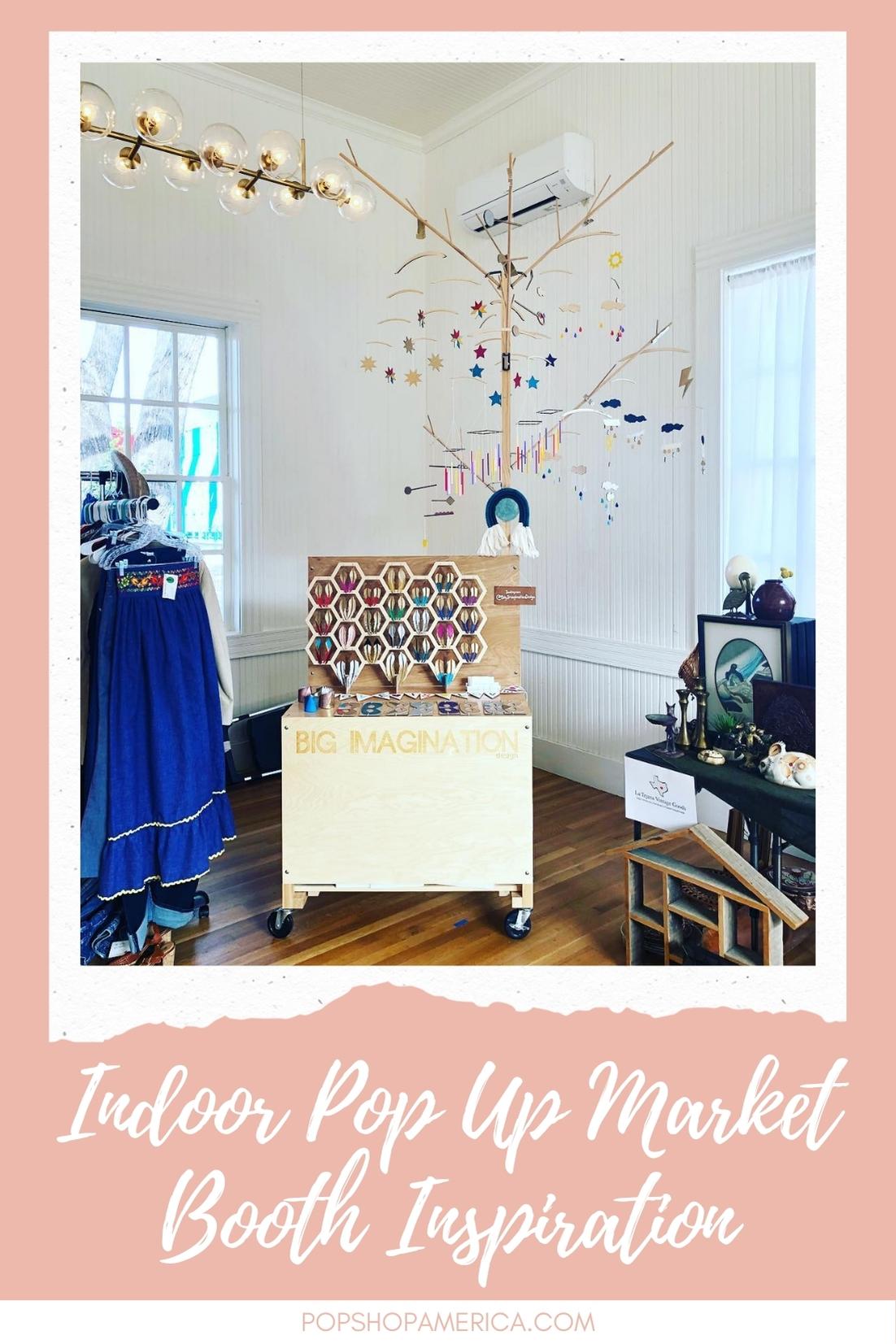This professionally taken photograph captures an indoor pop-up market booth with vibrant and eclectic decor. The image is framed by a pink triangle at the top and a white triangle around it, with text that reads "Indoor Pop-Up Market Booth Inspiration" at the bottom, followed by "PopShopAmerica.com" beneath. The store features white walls and brown hardwood floors, creating a clean and inviting space. To the left, a rack of clothes prominently displays a long, blue skirt, while on the right, a variety of smaller boxes and collectibles are positioned, including ornaments or earrings hanging from a decorative brown tree structure.

At the center of the image is a wheeled booth adorned with a honeycomb pattern, featuring the text "Big Imagination." The honeycombs appear to be filled with multicolored threads, adding a dynamic and creative flair. Above the booth, circular overhead lights illuminate the scene, and an air conditioner is visible in the background, hinting at a well-ventilated space. The color palette of the market includes blues, tans, whites, aquas, yellows, and reds, contributing to the overall lively and artistic atmosphere.